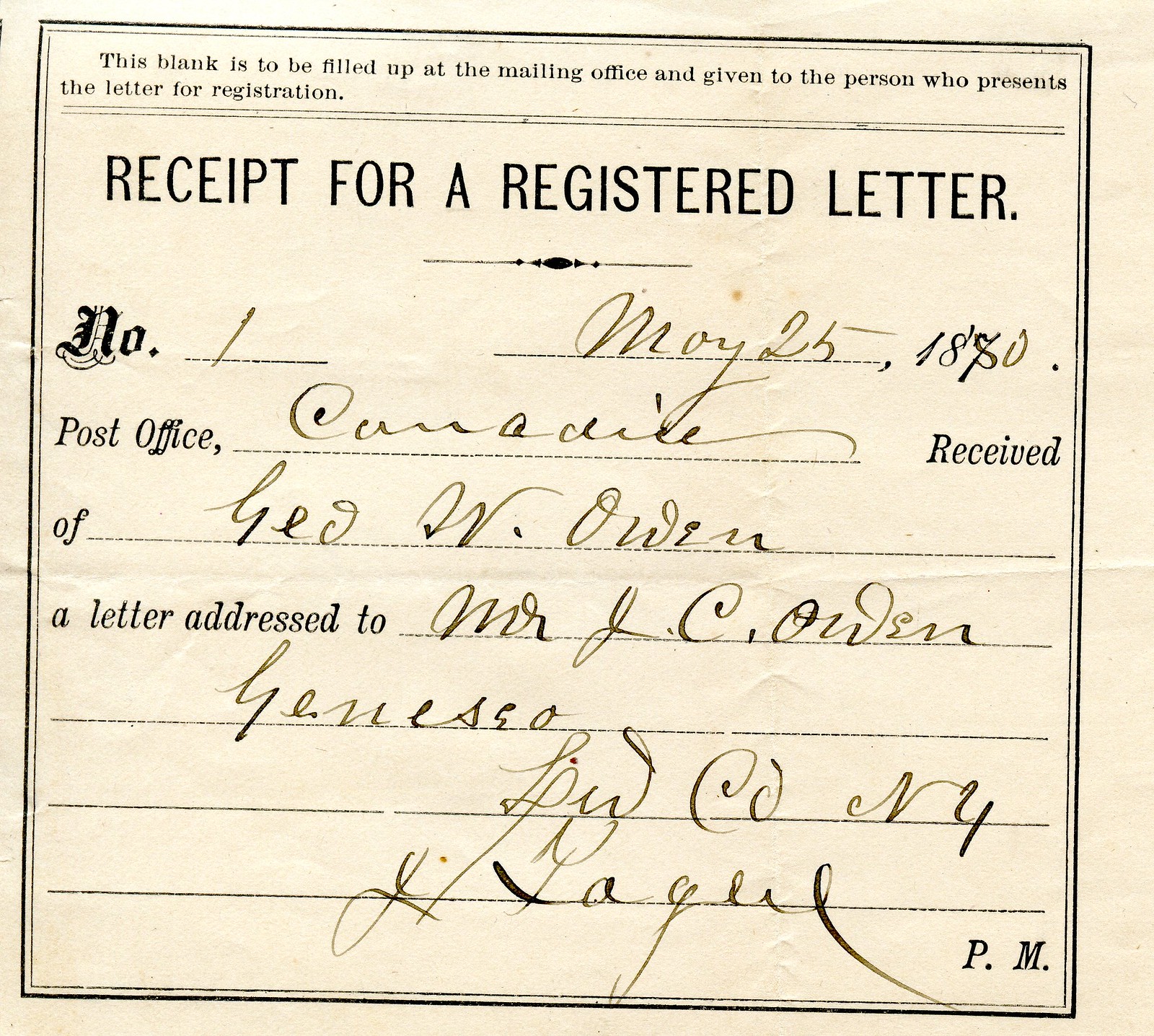This is an image of an old postal receipt from May 25th, 1870 or 1880. At the top of the receipt, it states, "This blank is to be filled up at the mailing office and given to the person who presents the letter for registration." This indicates it is a receipt for a registered letter. The receipt bears the number "1" written in ink. The post office name begins with a "C" and is faintly spelled out, possibly "C-A-R-R-A-D-I-L-E" or "Camachi," though it is difficult to decipher due to the aged and faint cursive ink. The receipt acknowledges the receipt of a letter from "G.E.O. V. Owen" or "Jed W. Owen" addressed to "Mr. J.C. Owen" in "Genesco" or "Janisa," "Lowe County, New York." At the bottom, there is a signature with the letters "P-M," likely indicating the postmaster.